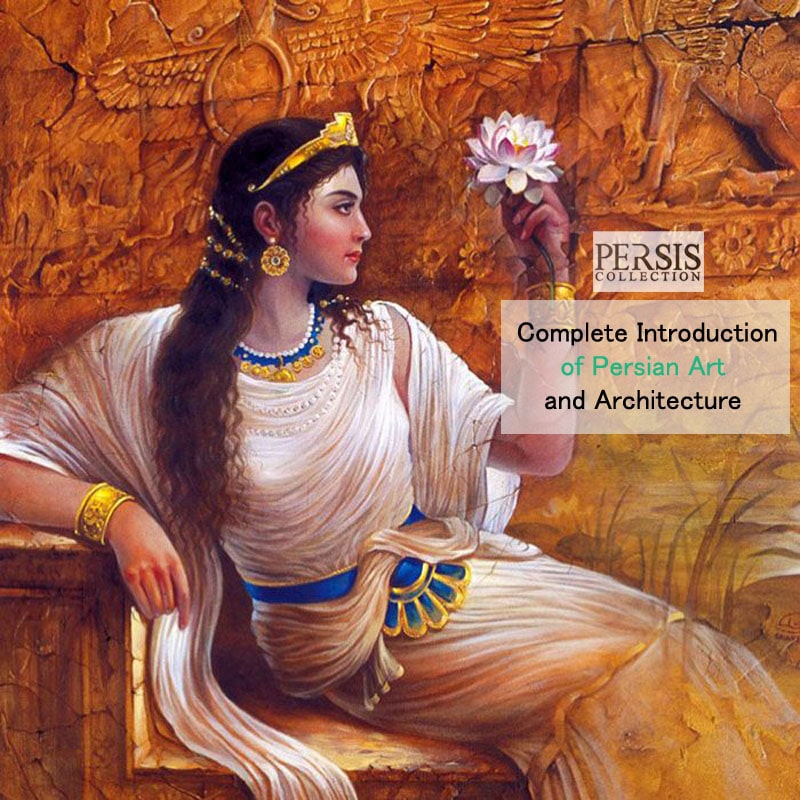This detailed illustration showcases an elegant Persian woman seated slightly reclined on a stone bench or throne, facing forward with her legs positioned to the right. She is adorned in flowing, white drapey robes reminiscent of a toga, highlighted with a blue and gold belt cinched around her waist. Her ensemble is complemented by a matching blue and gold necklace, an elaborate gold tiara, and gold bracelets on both wrists. 

Her hair is embellished with jewels, and she wears a striking earring. She holds a lotus flower delicately in her hand, gazing at it thoughtfully. The backdrop features an intricately carved stone wall adorned with figures, including what appear to be a lion, a bird, and possibly other animals or abstract forms, adding a historical and artistic depth to the setting.

To the right of the illustration are two white blocks of text. The first, smaller block reads "Persis Collection," while the larger block below it states, "Complete Introduction of Persian Art and Architecture," anchoring the artwork within a specific cultural and historical context. The overall color scheme of the painting is warm and golden, enhancing the ancient and opulent atmosphere of the scene.